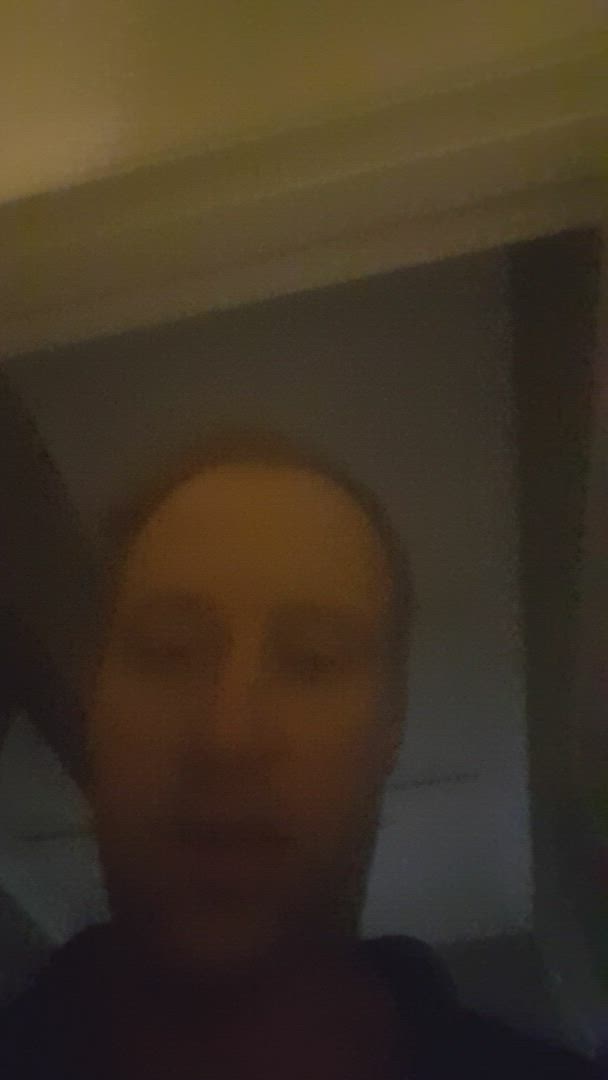This image captures a blurry selfie of a Caucasian male taken in low light, giving it a pixelated and low-quality appearance. The man appears to have accidentally taken the photo, as his mouth is open and he seems unprepared. His face, which is oval-shaped and has a noticeable forehead with short brown hair, is the main focus. Due to the poor image quality, his eyes and their color are unclear. He is dressed in a dark shirt, and only his upper neck and head are visible. The background consists of a gray ceiling or wall, a white wooden border at the top, and some dark elements on the side of his head. Overall, the photo is quite indistinct, with most details blurred and hard to discern.